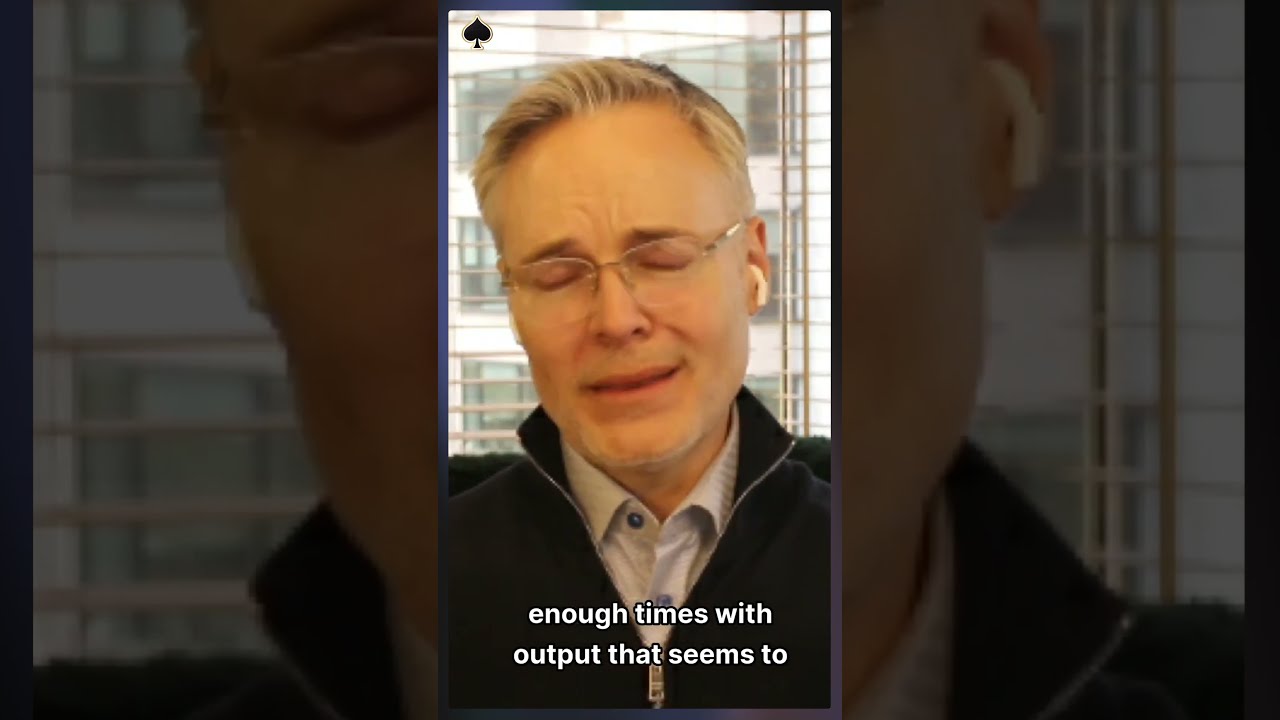The image is a vertical, cell-phone style picture of an older white man with a lighter skin complexion, centered from his upper chest to his head. The ambient lighting indicates it was taken during the daytime, as there is plenty of natural light coming through an open window with blinds. The man has short, white hair that is slightly raised in the front and swished to the side. He is wearing thin, silver-framed glasses and has an AirPod in his left ear. His eyes are closed, displaying a concentrated or possibly mid-sentence expression, with lines between his eyebrows and a mouth that appears partially open in a near-smile. He is dressed in a white and possibly blue collared button-up shirt, underneath a dark zip-up jacket with the collar raised. Superimposed in white text along the bottom edge of the image are partially readable words, suggesting it could be a screenshot from a video. The overall backdrop is a faded and zoomed-in version of the same picture, adding a frame-within-a-frame effect.